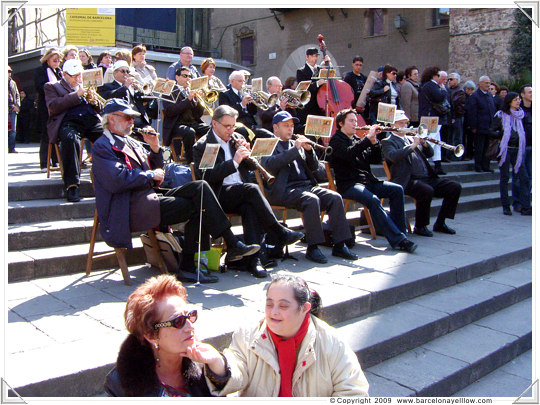The photograph captures a professional-looking orchestra or band performing outdoors in daylight on a series of stone or concrete steps. The orchestra, predominantly composed of middle-aged and older men dressed in formal wear, is arranged in two or three rows seated on wooden chairs. Musicians are engaged with various instruments like flutes, clarinets, trumpets, and possibly a cello, all reading from music sheets. In the bottom center of the image, two women stand out: one in a white jacket with a red scarf, touching the chin of the woman next to her, who wears sunglasses and has short hair. The setting is vibrant with an apparent sense of performance art, and onlookers gathered at the far right are gazing off, likely watching a live performance happening in front of the orchestra.